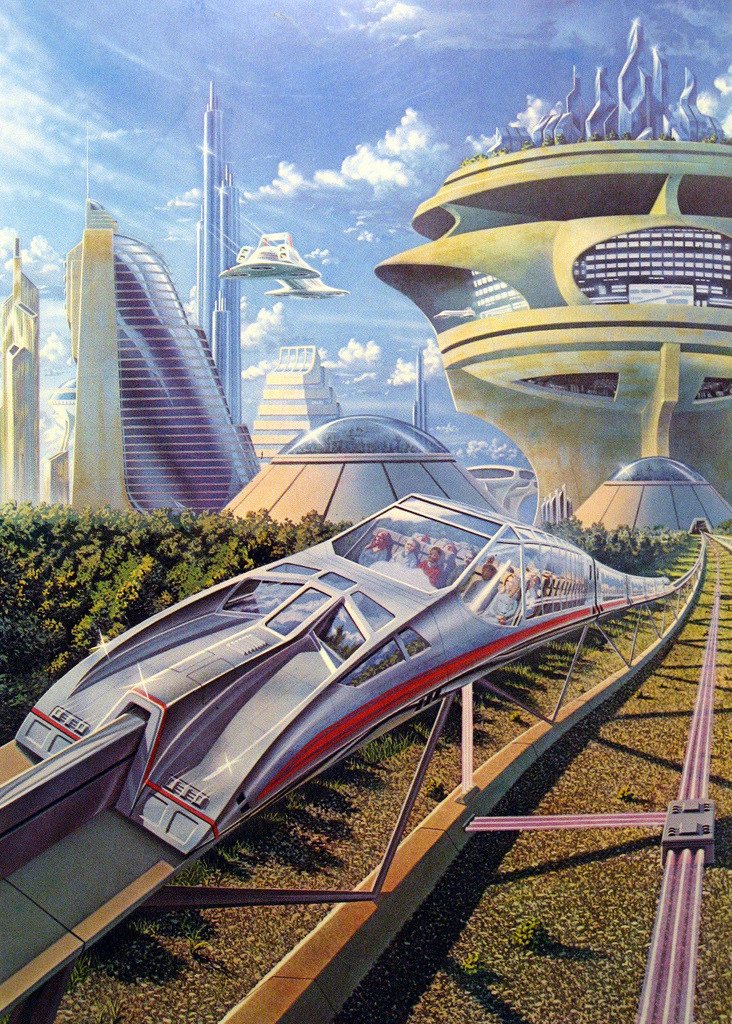The image depicts a vibrant, detailed painting of a futuristic world bathed in natural sunlight. The scene is dominated by a bright blue sky dotted with fluffy clouds, contrasting with the various dome-shaped and intricately designed futuristic buildings visible across the landscape. 

In the foreground, a sleek monorail reminiscent of a sports car glides along tall, electrified tracks. The train, which is primarily silver with a striking red stripe, has glass windows through which we see passengers seated and facing forward. The monorail, composed of about five cars, travels beside a lush field of plants. 

Above, flying ships and futuristic planes zip through the sky, adding to the scene's dynamic energy. To the left, green trees punctuate the landscape, with one particularly large dome-shaped building in the background featuring greenery on its rooftop. Additionally, a large roundish yellow building with silver spires offers a striking architectural focal point.

This multi-color artistic piece has no border or text, allowing the viewer to fully immerse themselves in this artist’s imaginative interpretation of a high-tech, utopian future.